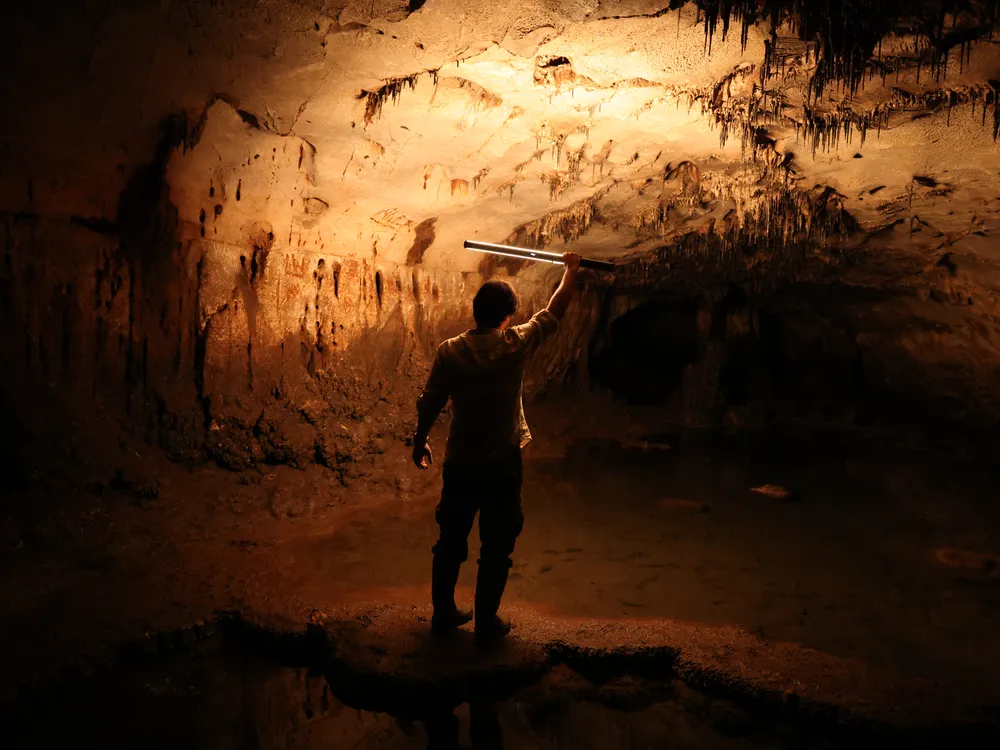In this image, a man stands in the depths of a dark cave, holding a sword-like light bar high above his head, which illuminates the cave's rough, reddish-brown interior. The rugged cave walls feature small stalactites hanging from the ceiling, and scattered rocks and patches of standing water can be seen on the muddy ground. The man, seen from behind, appears to be wearing a long-sleeve shirt with rolled-up sleeves, long pants, and possibly boots, although the dim light makes it hard to discern details clearly. A wristwatch seems to adorn his left wrist. He stands on a circular, natural stone platform, with the clear water reflecting parts of the cave's structure. The light he holds casts shadows, creating a stark contrast between the illuminated areas and the pitch-black surroundings, emphasizing the cave’s vastness and solitary atmosphere.